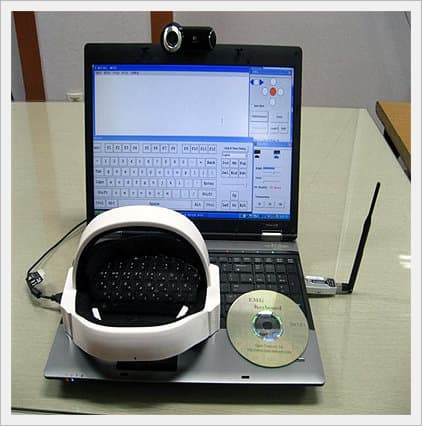The photograph captures a mid-2000s style laptop prominently positioned at the center on a bright white, shiny desk. The background showcases a white wall with two vertical brown boards on the left side, and an electrical outlet or jack visible beneath them. To the right edge of the image, there's a sliver of another desk or table, featuring light brown wood.

The laptop, open and powered on, displays a virtual keyboard and a blank text document on its screen. Additionally, a few virtual control buttons are visible. Positioned directly on the laptop's keypad is a small white motorcycle helmet with a black interior and a removed visor, resembling a virtual reality device. Adjacent to the laptop on the right, you'll find a CD with some labeling. A Wi-Fi dongle with a black antenna is plugged into the right USB slot of the laptop, and a black webcam with a silver circle adorns the top of the laptop screen.

The scene likely depicts an office setting, possibly engaged in testing hardware, as suggested by the various connected devices and accessories. The color palette includes touches of silver, white, black, red, and blue, contributing to the detailed and somewhat technical atmosphere of the workspace.